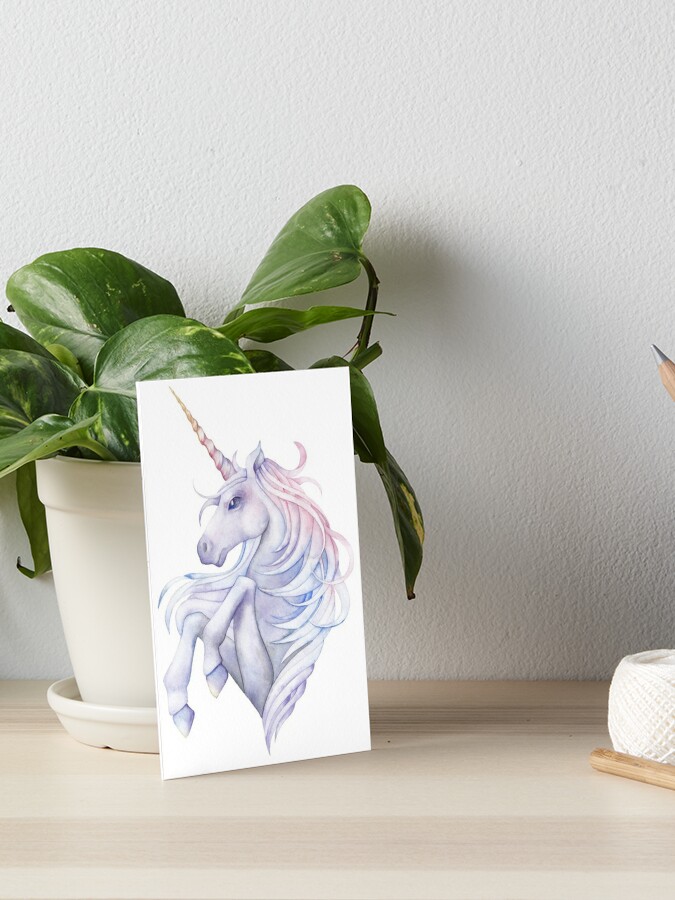The photograph showcases a vibrant setting featuring a potted indoor plant on a light birch-colored wooden surface against a white textured wall. Leaning against the plant pot, which is cream-colored, is a white card displaying an artistic rendering of a unicorn. The unicorn illustration is detailed with a periwinkle purple body and a mane that transitions beautifully from pastel pink to blue and purple. The horn has a striking gradient from a pink base to a golden tip. The plant boasts large, waxy green leaves with a hint of yellow variegation. To the right of the unicorn card, a ball of twine rests adjacent to a small brown stick, and just barely visible on the far right edge is the sharpened tip of a pencil.